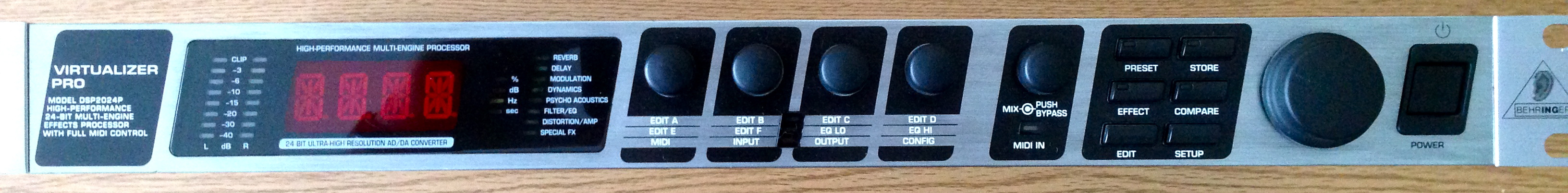This image depicts a piece of sound equipment, possibly a synthesizer or audio processor, called the "Virtualizer Pro." The device spans the entire width of the photograph in a long rectangular shape. Its casing is silver metal, and it rests on a light wood surface. On the far left side, there's a skewed black square featuring the name "Virtualizer Pro" in white text. Next to this is a black rectangular screen that displays a red box with four red zeros, indicating the device is currently powered off. 

Following the display are four black dials labeled Edit A, Edit B, Edit C, and Edit D, each set within its own small black rectangle. There's then a gap, followed by an additional similar dial. Proceeding to the right are six small black rectangular buttons arranged in two rows of three. Next to these buttons is a larger black circular dial, likely used for volume control, and finally, on the far right, there's a black square button functioning as the power switch.

The detailed layout, including the specific placement of dials and buttons, along with the intricate text and labeling, suggests its use in complex audio processing or music creation. The entire unit is outlined with a wood-grain finish, adding a classic touch to its modern functionality.